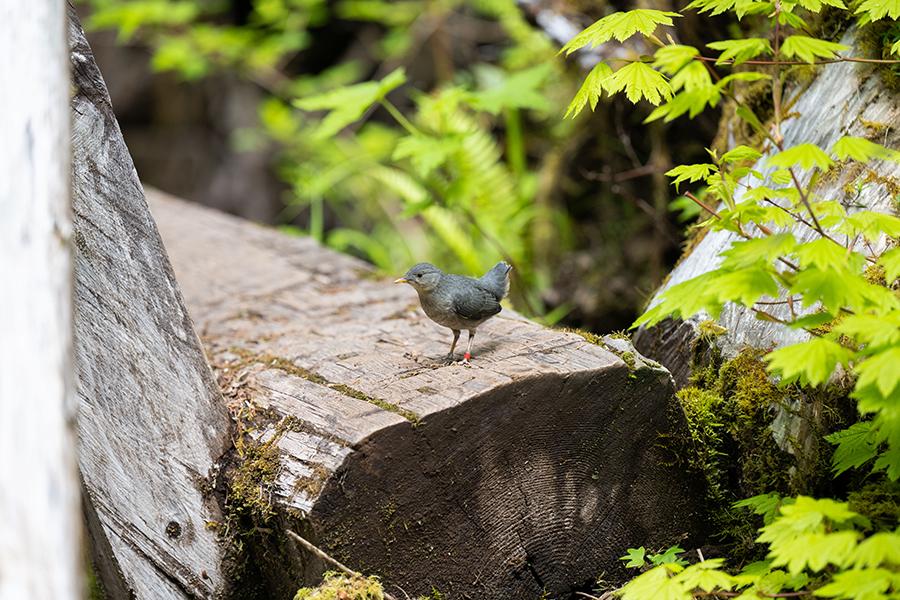This captivating photograph captures a lone, small gray bird perched on a large, sawn-off log, deep within a forest teeming with life. The bird, which features a yellow beak, a tiny black eye, and a distinct red tracking band on its left leg, stands prominently against the brownish-gray wood. The foreground presents the bird and the partially sawed tree with remarkable clarity, while the background, though blurred, reveals a rich tapestry of light green spring leaves, potentially from maples. Moss drapes over parts of the trees, adding a lighter green hue, and ferns peek through a dense thicket, suggesting a lush and thriving woodland environment. Bright and diffuse lighting, indicative of mid-morning or an early afternoon, enhances the natural beauty of this serene forest setting.